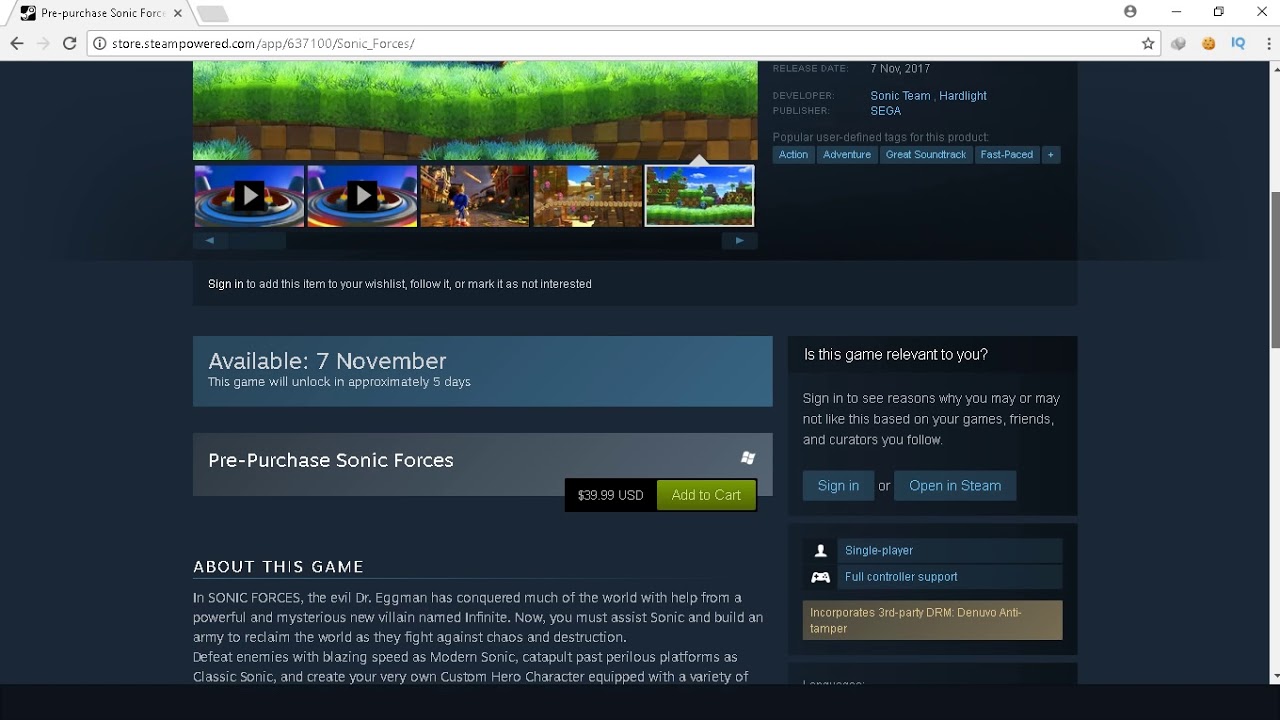This screenshot captures a store page on the Steam platform, showcasing a pre-purchase listing for the game *Sonic Forces*. The page prominently displays the game’s release date, set for November 7, 2017, with a note indicating that the game will unlock in approximately 5 days, suggesting that the screenshot was taken around November 2, 2017. *Sonic Forces* is priced at $39.99 USD, and there is a clearly visible "Add to Cart" button for users to proceed with their purchase. The platform is confirmed to be for Windows, as evidenced by the Windows logo on the page. Detailed descriptions about the game’s storyline and features are provided, mentioning key elements such as single-player mode, full controller support, and the inclusion of third-party DRM. Overall, this page offers comprehensive information for potential buyers ahead of the game's official release date.